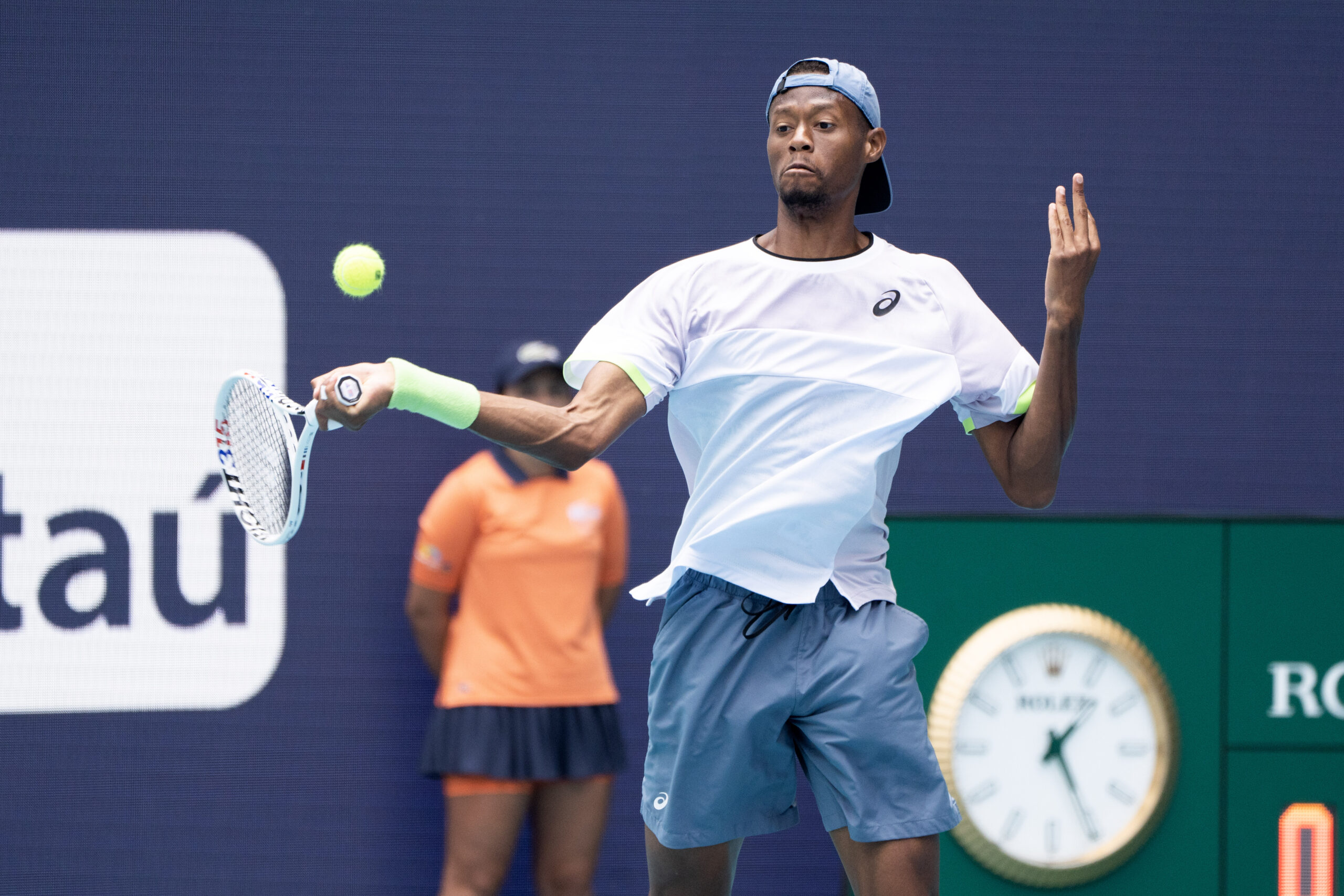This color photograph captures professional tennis player Chris Eubanks, an African-American male, mid-action as he prepares to hit a green tennis ball with his right hand using a white tennis racket marked by black, red, and blue text. Eubanks is donned in a white athletic top adorned with a black ASICS logo on the upper left, and blue athletic shorts that fall just above his knee, featuring the same ASICS logo in white on his right leg and black tie strings in the middle. His ensemble includes a backward blue baseball cap and a green wristband on his right wrist. The backdrop consists of a bluish-purple hue with visible details: a green Rolex advertisement featuring a clock with a gold rim on the lower right side, and a rounded white rectangle with the letters "TAU" on the left. Additionally, a woman in the background, dressed in an orange top, a navy blue skirt with orange compression shorts, and a blue hat with a white emblem, adds to the dynamic scene. The image meticulously captures both the athletic prowess of Eubanks and the vibrant environs of the tennis event.